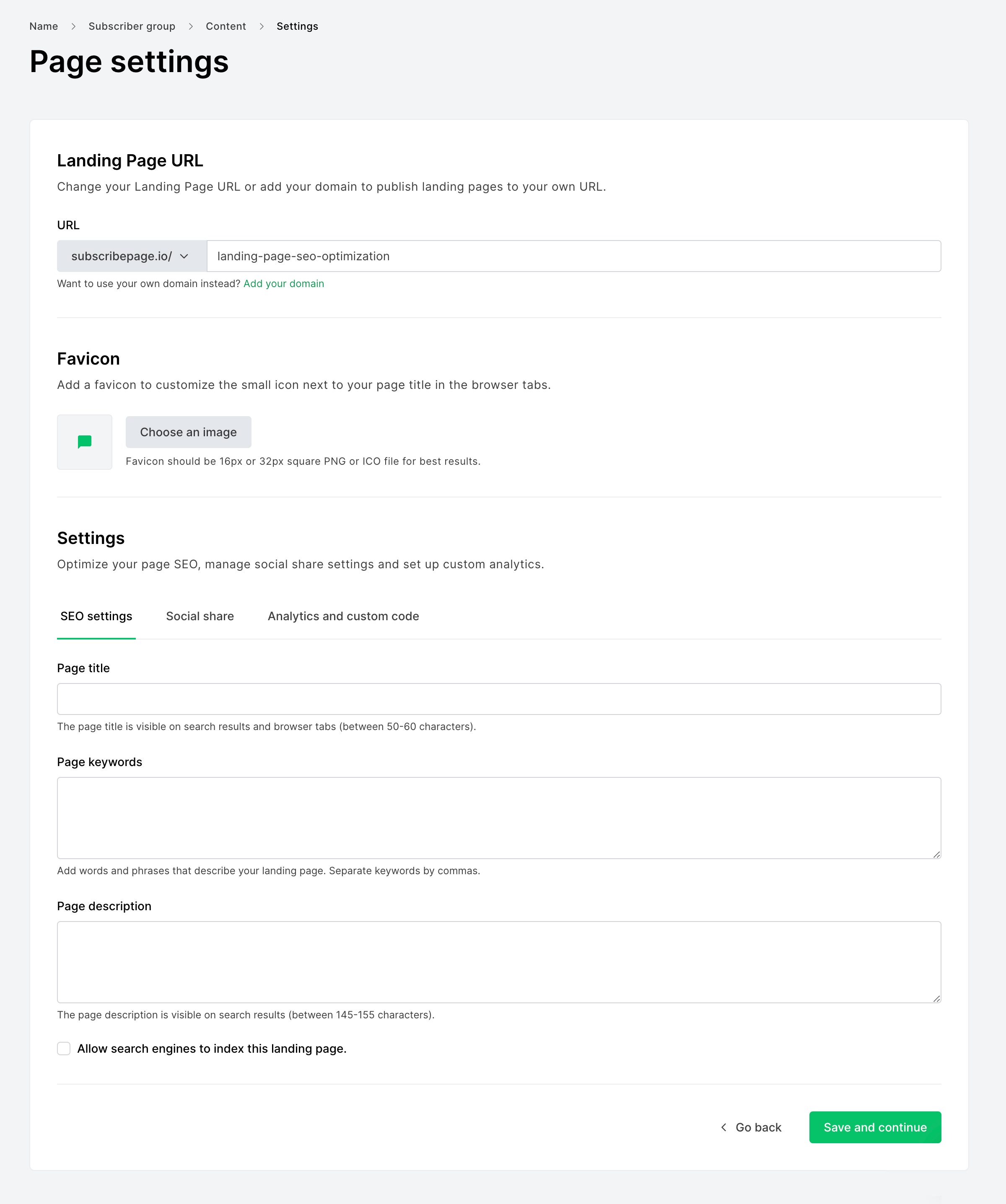In this image of a website builder interface with a light smoke gray background, various settings and customization options are prominently displayed. At the top of the interface, there are four tabs labeled "Name," "Subscriber Group," "Content," and "Settings." Below these tabs, bold black text reads "Page Settings."

A large white square within the gray background houses several specific options for configuring the landing page. In the top left corner of this white square, the text "Landing Page URL" appears, followed by a description that reads, "Change your landing page URL or add your domain to publish landing pages to your own URL." Below this is a section where users can input a URL.

Further down, an option labeled "Favicon" allows users to add a small icon next to their page title in browser tabs. A button is present to choose and upload an image for the favicon.

Additionally, there are settings for optimizing the page's SEO, managing social share settings, and setting up custom analytics. This section includes three tabs: "SEO Settings," "Social Share," "Analytics," and "Custom Code." Users can enter the "Page Title," "Page Keywords," and "Page Description" in the provided fields. There is also a checkbox to enable search engines to index the landing page.

At the bottom right of the interface, buttons labeled "Go Back" and "Save and Continue" provide options for navigation and saving changes.